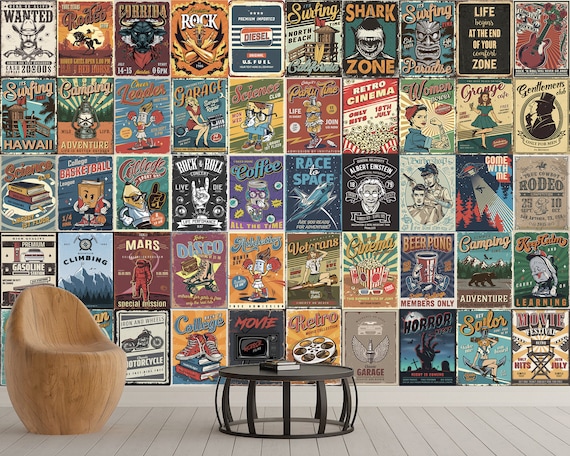The photograph showcases a room with distinctive decor. Dominating the background is a wall entirely covered in 50 perfectly aligned, rectangular posters. These posters span various themes and styles, resembling vintage advertisements or comic book covers. They feature an array of vivid colors and intriguing subjects, such as "Wanted" posters, pin-up girls, rock concerts, horror movies, surfing scenes, coffee ads, and more. Titles like "Shark Zone," "Rock," "Rodeo," "Disco," "Mars," "Race for Space," and "Garage" indicate the eclectic mix. At the bottom right, a "Movie Festival" poster can be spotted. The posters are uniformly sized and spaced, creating the impression of a custom wallpaper.

In the foreground, the room features white wooden slat flooring. Centrally placed is a black, cylindrical coffee table with bended posts along its sides, resembling a drum bass. Two books rest atop this table. To the left, there's a uniquely carved wooden chair without armrests, designed with a simplistic, rustic appeal. The overall composition of the room merges retro and eclectic elements, creating an inviting and intriguing visual story.